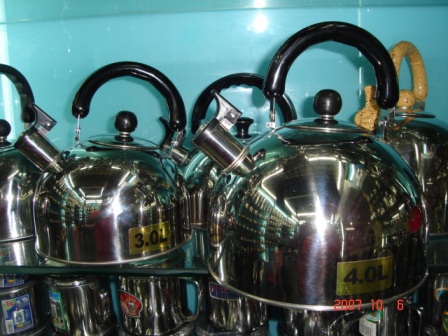This image showcases an arrangement of stainless steel tea kettles displayed on a glass shelf against a vibrant light teal blue wall, likely in a store setting. Each kettle features a highly reflective, dome-like structure with curved black handles, except for one in the back right, which is distinguished by a light tan handle with brown specks. The kettles are labeled with gold squares indicating their capacities in black text, specifying 3.0 liters on the left and 4.0 liters on the right, positioned at the front bottom of each kettle. Reflective surfaces capture the flash from the camera. Below the main display is a partially visible row of other steel kettles, possibly of a different shape or function. An old photo stamp reading "2017-10-6" is seen in the corner, adding a dated aspect to the setting.